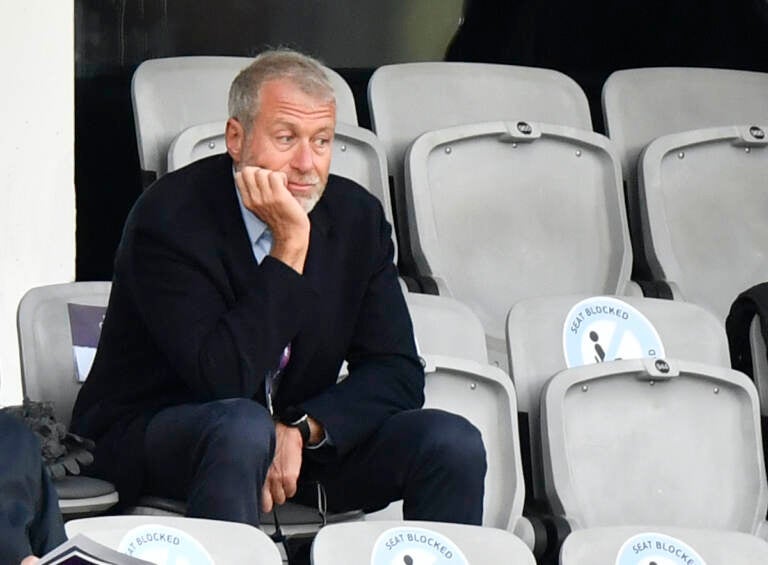In this image, an older Caucasian man with grey hair and a slight white beard is seated in what appears to be stadium seating, possibly during a sporting event. He wears a black overcoat and a blue button-up collared shirt, paired with dark blue jeans. A black smartwatch adorns his left wrist, and a purple lanyard hangs from his neck. The man rests his right elbow on his right knee, supporting his chin on the palm of his right hand, looking somewhat bored or contemplative as he gazes off to the side.

The grey plastic seats surrounding him are mostly empty and feature signs indicating they are blocked for seating, likely for social distancing during the COVID-19 pandemic. Some personal items, such as gloves or possibly a shirt, are placed on the seat beside him. Behind him, a glass barrier suggests the presence of a higher-end seating area, possibly a VIP section. This overall scene hints at a socially distanced event, with the man sitting alone amidst multiple rows of vacant seats.